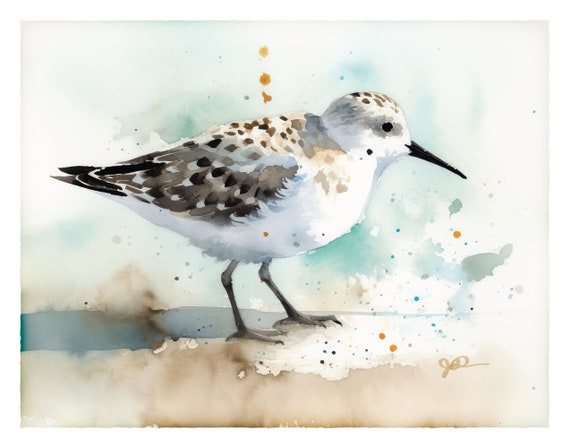This is a detailed watercolor painting of a small bird. The bird is primarily white with an underbelly and chest that are distinctly white. It has a long, black beak pointing slightly downward to the right. Its eyes are black and round. The bird's wings and back display a mix of brown, gray, and black speckles and dots, with noticeable splotches of white. Its legs are grayish-charcoal with black talons, and it stands on an abstract base that combines white, blue, brown, and beige colors. The background features an abstract, sky-like quality with aqua and white hues resembling clouds. There are speckles of various colors, including yellowish-brown, blue, and black, scattered throughout the image. Notably, three yellow-brown specks are aligned in a row above the bird. The painting is signed by the artist in the bottom right corner, though the signature is not clearly legible. This piece captures the delicate and ethereal nature of the scene through its soft, blending watercolor technique.